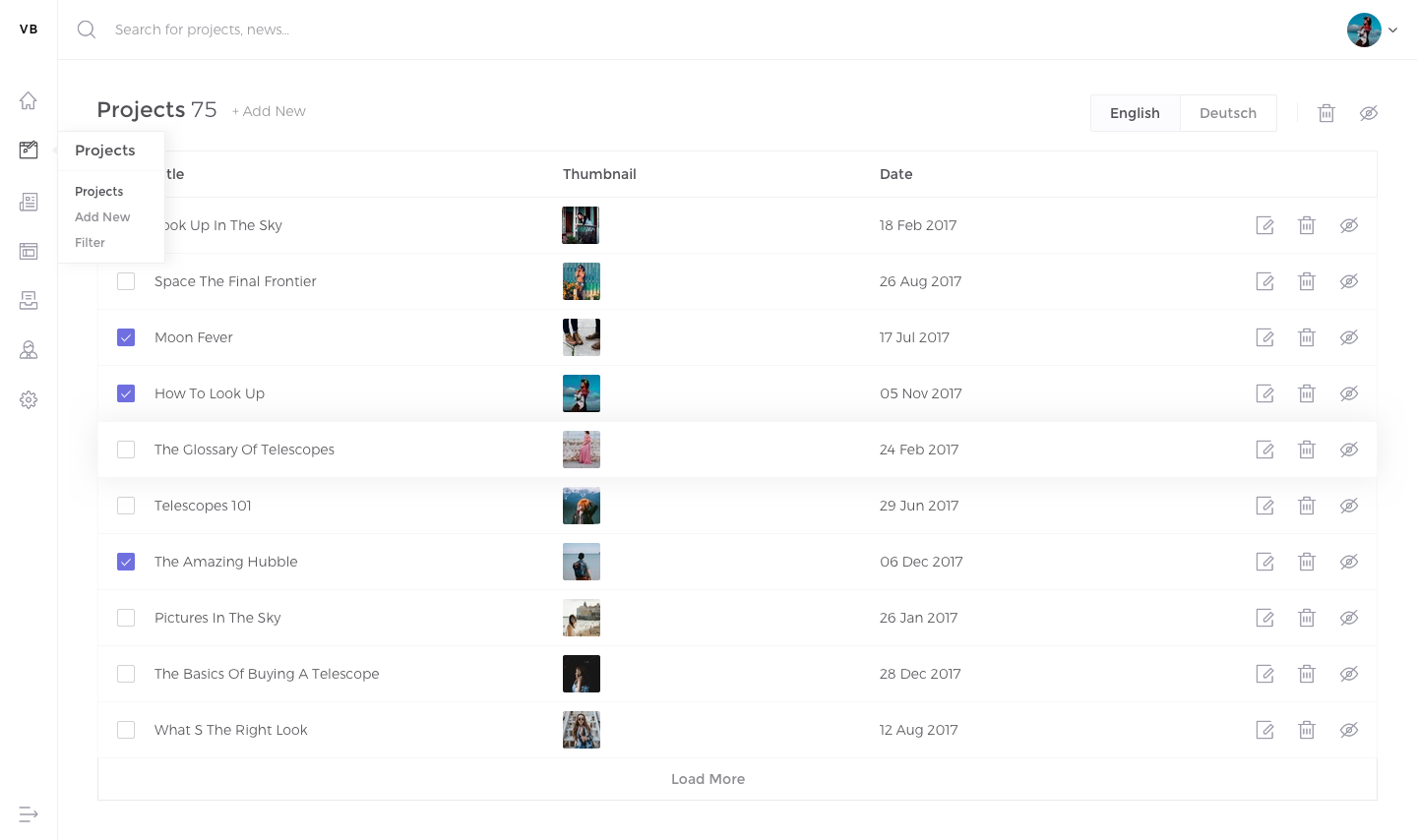This screenshot showcases a cropped view of a content management or project management tool with a clean white background. The interface prominently displays a list of active projects with an option to add new ones, capable of managing tasks, calendars, reports, and user profiles. 

At the very top left corner, a bold "VB" logo is visible, immediately followed by a search bar labeled "Search for projects, news" in small gray letters. In the far top right corner, a circular user profile photo accompanied by a dropdown icon is positioned.

Directly below this top navigation strip, the word "Projects" appears in bold black font, followed by the number "75" and a small gray "Add New" link to the right.

On the far left side, a vertical strip of small icons is presented. The first icon represents a home symbol, while the second icon, resembling a piece of paper, is highlighted with an open dropdown containing the word "Projects," indicating that the project management view is currently active.